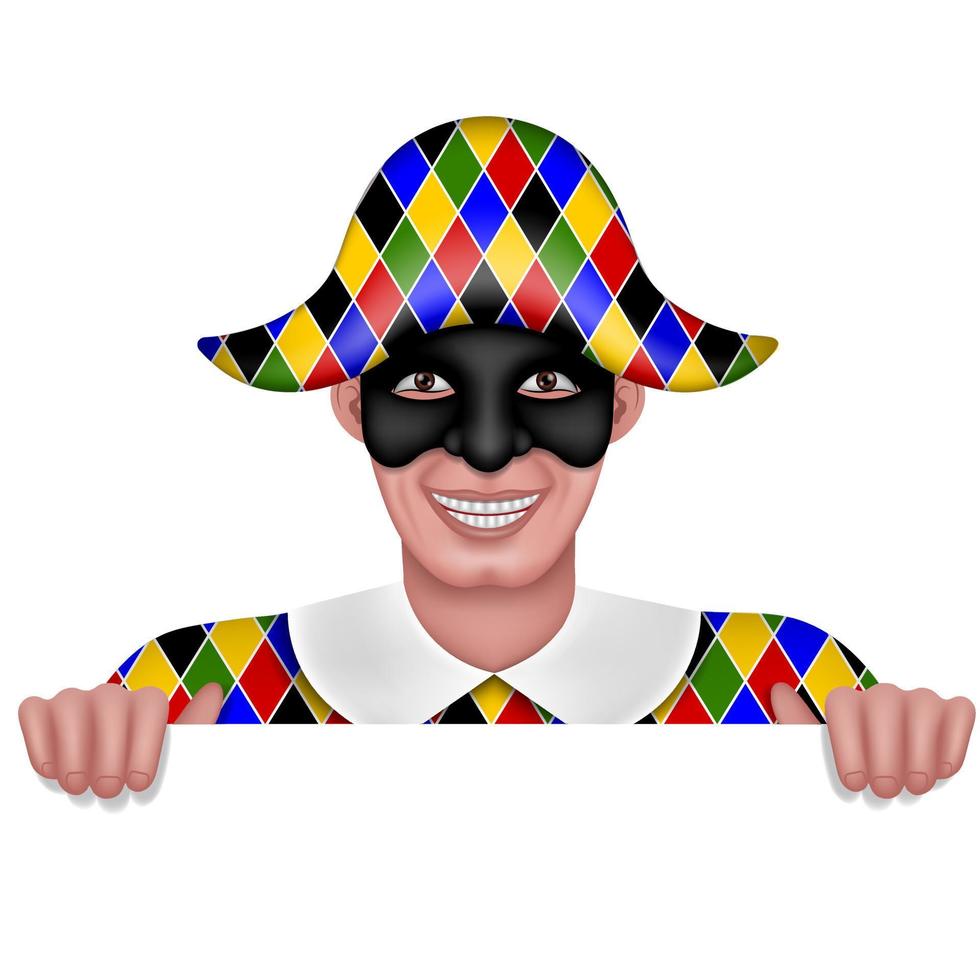This image is a detailed cartoon drawing of a jester character appearing to pop out of a box, with a detailed and vibrant style. The jester is wearing a multicolored diamond-pattern suit in green, red, black, and yellow, complemented by a large white collar. His uniquely shaped hat, which appears oval at the top and spiky at the sides, also shares this intricate diamond pattern. The jester's white-gloved hands are folded over the edge of a white surface, giving the impression that he’s either holding onto or climbing over something. His face is partially concealed by a black eye mask that covers his nose and eyes, revealing his big brown eyes filled with a mischievous spark. He sports a broad, toothy smile with teeth resembling little chiclets, adding a slightly eerie quality to his expression. His skin is very pale, enhancing the contrast with his brightly colored outfit. Overall, the dynamic posture and rich details make the character stand out vividly against the plain background.